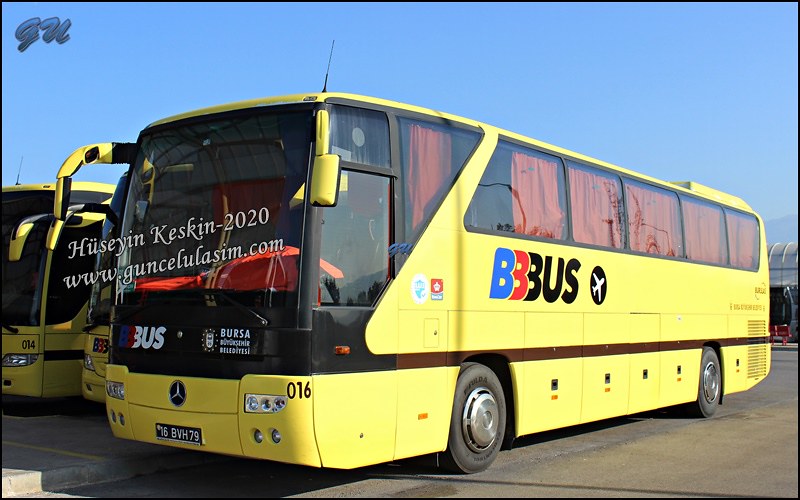This is a detailed photograph showcasing multiple bright yellow Mercedes buses. The primary focus is on a front-and-center bus, viewed from an angle that captures both its front and right side, set against a clear blue sky. The bus prominently displays a large Mercedes emblem on its front bumper. Emblazoned on the side of the bus is the text "BBBUS," with the triple B's in blue, red, and black respectively, followed by a black capital "US." Adjacent to this text is a black circle featuring a white airplane icon angled at about 45 degrees. The bus, with large tinted windows and orange curtains, has the identification number "016" on its front right corner. Written across the front windshield is "Hussain Keskin 2020" along with a URL, www.gunsalulahsim.com, in a foreign script. Mirrored assemblies protrude from the driver's area, framed by yellow armatures. The buses rest on a concrete surface, part of a parking lot with several other similarly colored buses in the background. Additionally, there is a building with a glass roof visible further in the background.